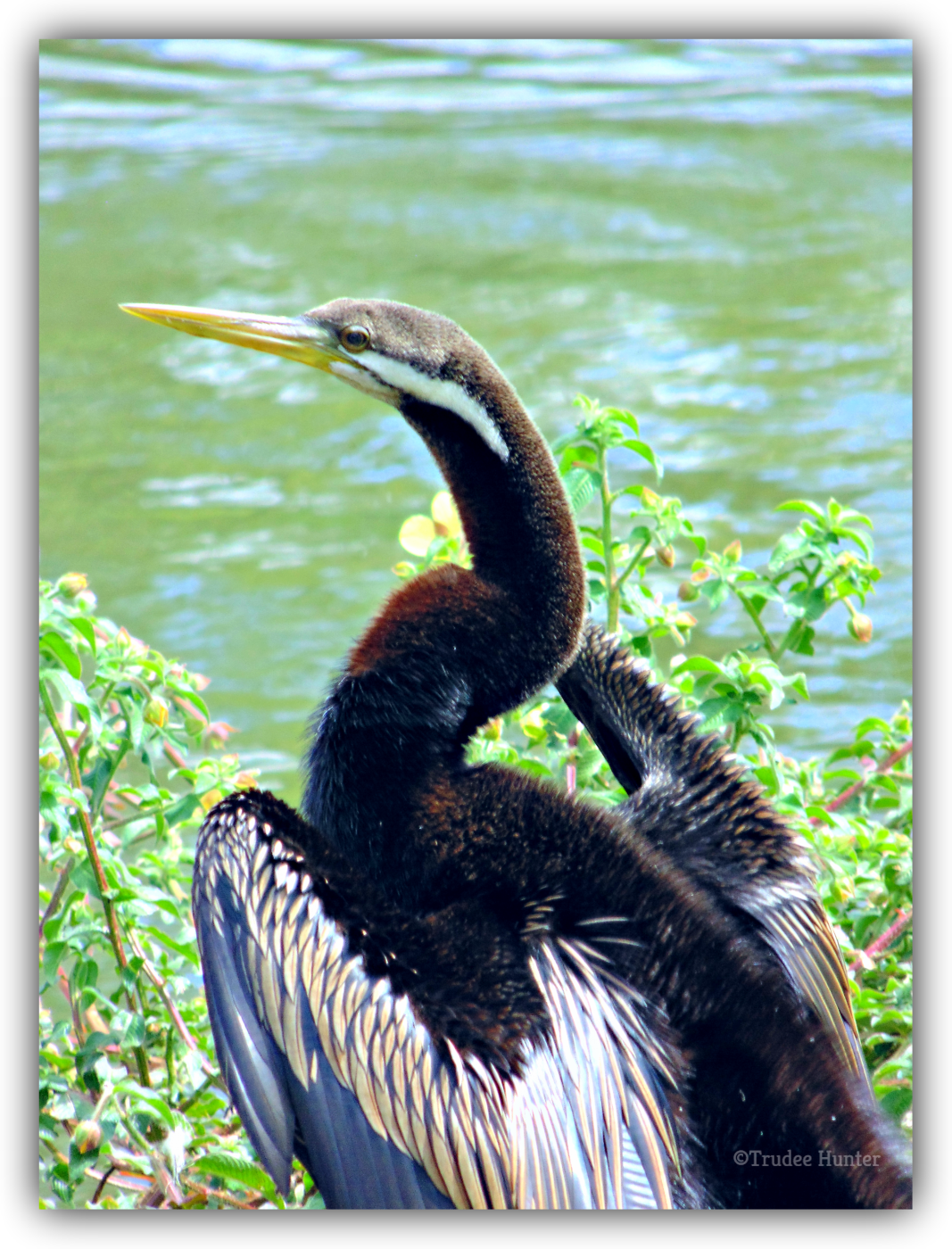This product photograph features a rectangular poster with a breathtaking image of a distinctive bird. The poster, designed to be displayed on a flat white surface to highlight the product for online listings or catalogs, depicts a black bird with a long, fuzzy neck and elegant white feathers on its wings. This striking bird bears a resemblance to a swan but is also likened to a heron or kingfisher in terms of its dark feather patterns and a long yellow bill. The bird, which also has lighter feathers on the top of its head and white feather details running from underneath its eye down its neck, is captured looking to the left amidst what appears to be an outdoor daytime setting. Surrounding the bird are green plants and shrubs, with a greenish body of water visible in the background, adding to the natural, serene ambiance of the photograph. The poster includes a semi-transparent watermark in the bottom right corner that reads "Copyright, Trudee Hunter," ensuring the artist's name, spelled T-R-U-D-E-E H-U-N-T-E-R, is distinctly recognized.